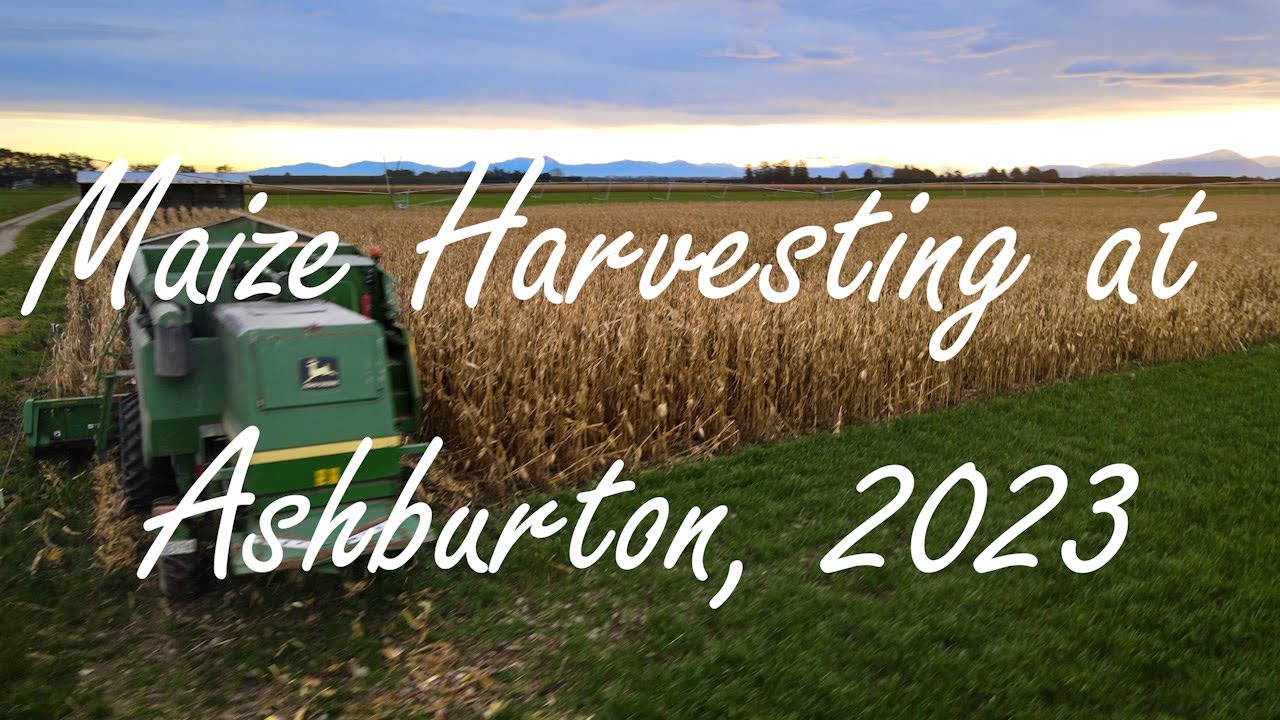The image captures a scenic agricultural scene under a cloudy sky that transitions from a blue-gray tan in the upper half to clearer skies at the bottom. Dominating the background is a blue mountain range that fades to gray on the right-hand side, where a line of trees stands tall in front. Below the mountains, there are expansive fields: a brown-tan farm field indicating dried maize plants, adjacent to a lush green field. A long rectangular shed marks the edge of the fields.

In the foreground, a John Deere harvester, painted a distinct green with a boxy front and large blade at the rear, is moving from the tan maize field into the green grassy area. The harvester's bold green hue and the recognizable John Deere logo are prominently visible. Long water pipes stretch across the green field, hinting at irrigation efforts. This is complemented by a dirt road to the left, providing access around the fields.

Text overlaid on the image reads "Maize Harvesting at Ashburton 2023," clearly identifying the scene's context. This image captures the diligent harvesting process, showcasing both natural and agricultural elements in perfect harmony.